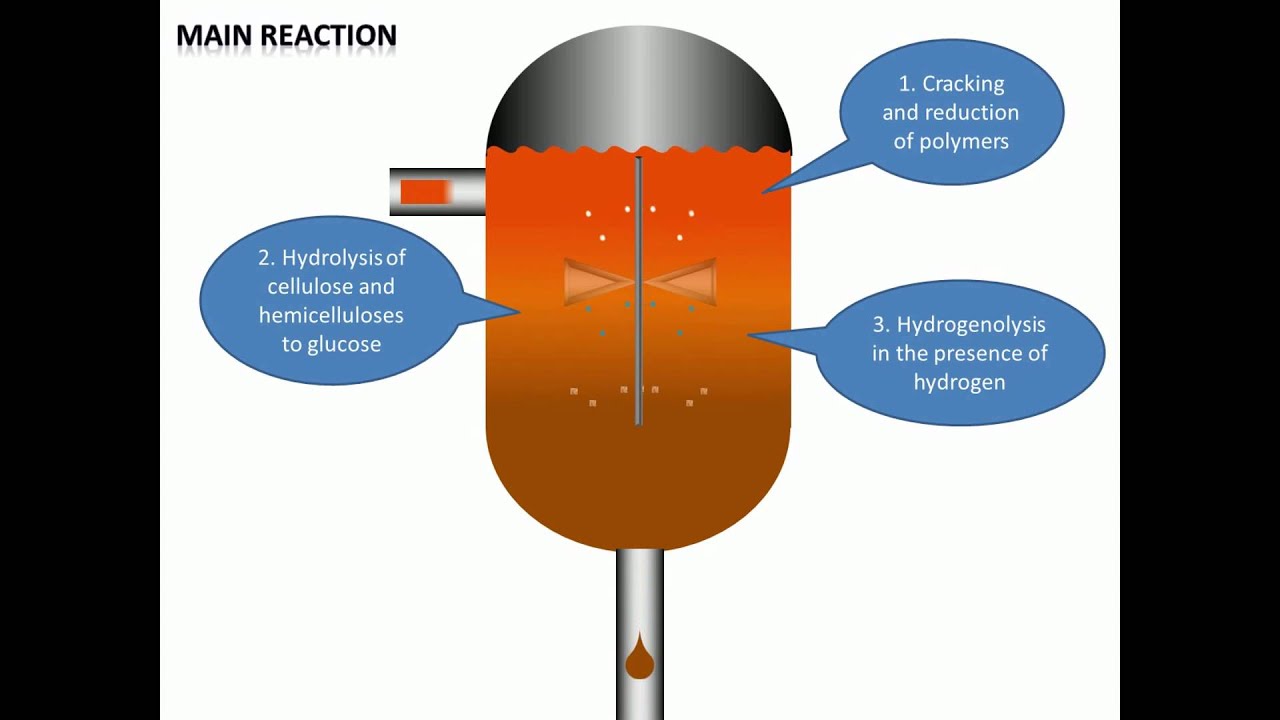The image is a detailed scientific diagram labeled "main reaction" in the upper left corner. The central focus of the image is an oblong, capsule-like object with a silver top and a gradient of orange to brown hues at the bottom. The background is white, bordered on both sides by vertical black lines. From the bottom of the capsule extends a silver tube, from which a drop of the orange liquid appears to be falling. Additionally, another silver tube is connected to the upper left side of the capsule. 

Three blue speech bubbles provide detailed explanations of the stages involved in the chemical process. The first bubble, located at the top right, reads "cracking and reduction of polymers." The second, situated to the middle left, states "hydrolysis of cellulose and hemicelluloses to glucose." The third is found in the center right, declaring "hydrogenolysis in the presence of hydrogen." This comprehensive diagram illustrates a sequence of chemical reactions, highlighting various stages of a complex scientific process.